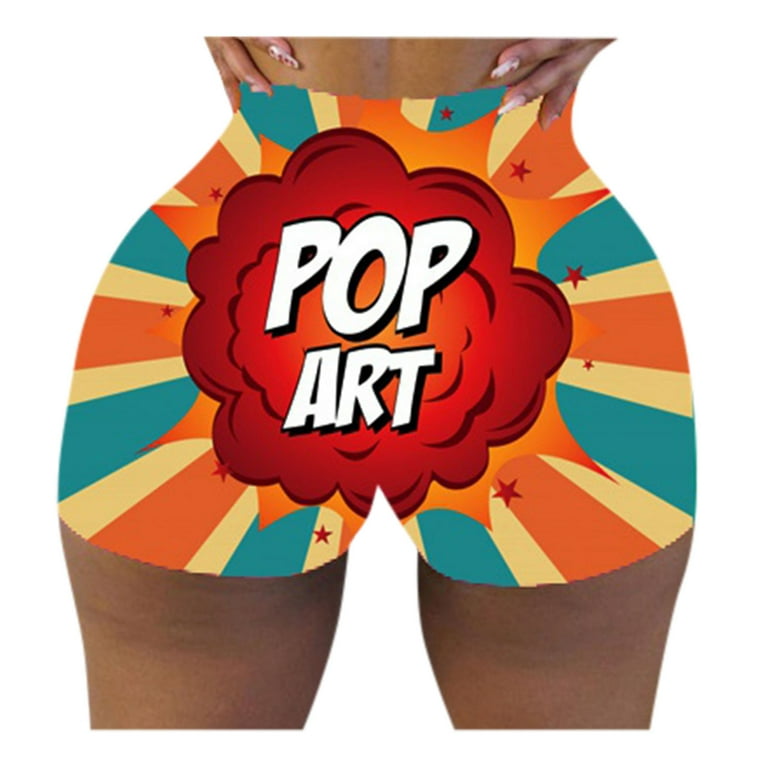The image depicts the backside of a woman with brown skin, likely African-American, whose hands are positioned around her waist, with her fingernails visible above her buttocks. The woman appears to be wearing digitally superimposed underwear. The design of the underwear features a large, red cloud at the center with the words "POP ART" in white lettering, outlined with black shading. This red cloud is encircled by an orange starburst, from which additional reddish stars radiate outward in various directions. Further decorating the undergarments are stripes in teal, light yellow, and orange that expand towards the edges of the woman's silhouette, creating a vibrant and dynamic explosion effect.